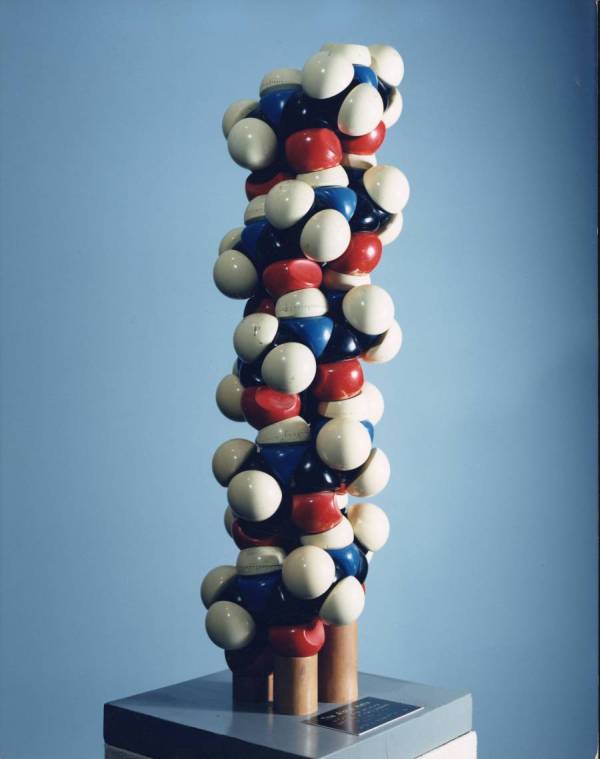The image features a tall, intricate art object representing a molecular structure, possibly symbolizing DNA or another scientific concept. The structure is composed of interconnected spheres in four colors: white, blue, red, and a less noticeable black. These spheres cluster together, forming a vertical, stick-like formation. The model is supported by four cylindrical wooden stands at its base. This entire assembly is positioned on a sturdy, square-shaped gray pedestal, which has a small black plaque with unreadable text affixed to it, likely providing a description of the object. The background of the image features blue walls that gradually darken towards the edges, creating a gradient effect.